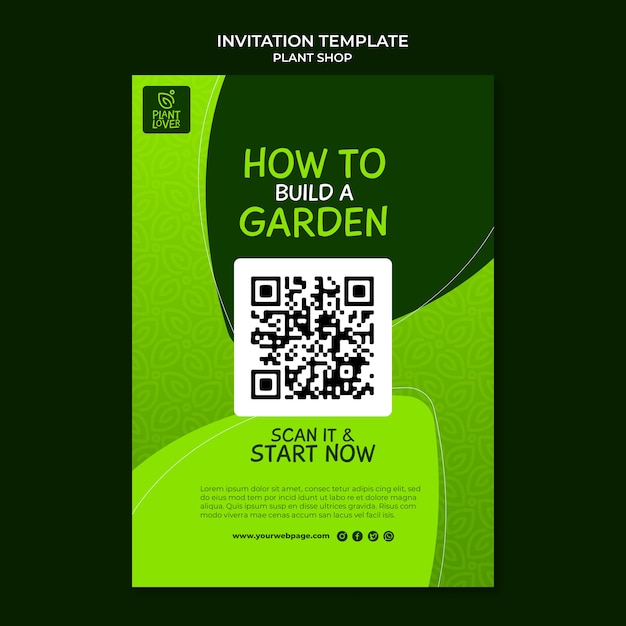The image depicts an advertisement template primarily designed for a plant shop. It features a sleek, black background with white text at the top labeling it as an "Invitation Template" for a plant shop. The central section of the image is dominated by various shades of green, ranging from neon to dark, adorned with a flowery and leafy design. In the upper left corner, there’s a logo labeled "Plant Lover," and prominently in the center, the title reads "How to Build a Garden." Below this title, there’s a QR code with an adjacent instruction that reads, "Scan it and start now." The bottom of the image includes several small black circles containing social media icons and a placeholder text "www.yourwebpage.com.” The template is designed to be customizable for different themes or businesses, such as a boat shop using blue shades, making it versatile for various types of event advertisements. The very small text beneath the QR code is likely containing additional instructions or terms and conditions.